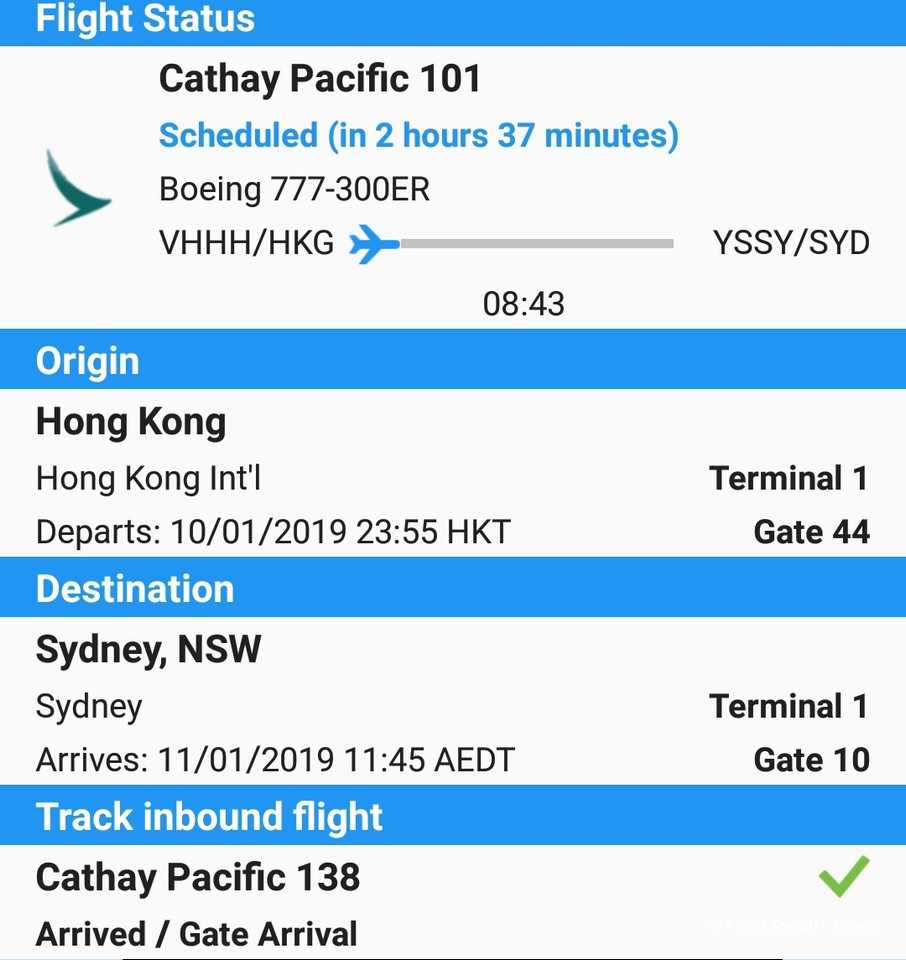A detailed caption for the given image could be:

---

A smartphone screenshot displaying flight status information. The screen is slightly taller than it is wide, characteristic of mobile displays, but not in the usual ratio. The interface features four blue bars spanning the width of the screen, labeled in white text as "Flight Status," "Origin," "Destination," and "Track Inbound Flight." Below the "Flight Status" bar, the text reads "Cathay Pacific 101," indicating the flight is scheduled to depart in 2 hours and 37 minutes. It shows the aircraft as a Boeing 777-300ER. Below this information, there are various numbers and an airplane emblem, suggesting a progress tracker for the flight. This section also displays the number "843." An icon on the left, possibly an advertisement, is visible.

Under "Origin," the text lists "Hong Kong," providing details such as the gate, terminal, and departure time. The "Destination" section indicates "Sydney, NSW," along with the arrival time, date, terminal, and gate. This bar also includes the flight number and status, confirming if the flight has arrived.